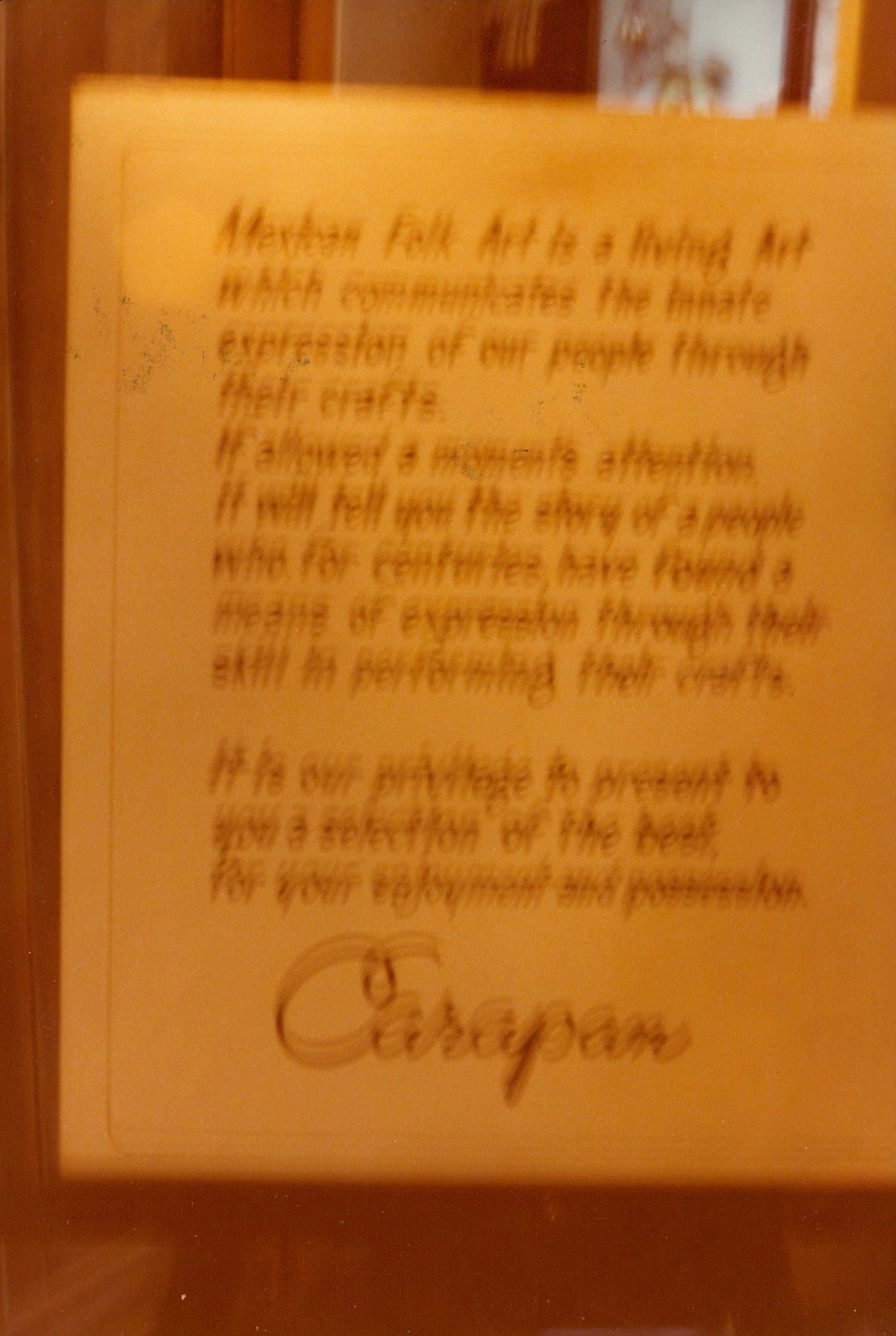This photograph captures a blurry image of a piece of writing on beige paper. The handwriting appears to be in a script or cursive style, and though the text is mostly illegible, the word "art" is intermittently discernible. The ink used is a dark brown or possibly gold hue. The paper seems to be a page from a book. The setting appears to be an indoor room with medium brown hardwood doors and lighter brown hardwood floors visible in the background, suggesting a cozy, residential environment.